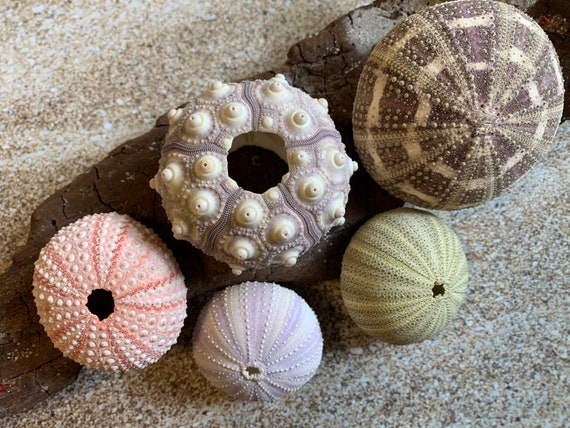This full-color, square photograph, likely taken outdoors under natural light, captures a detailed arrangement of five roundish marine creatures, possibly animals or shells, resting on a flat, brown and gray rocky surface. The creatures are organized with three on top and two on the bottom. Starting from the bottom left, there is a primarily white and pink shell with darker pink stripes radiating from a central hole. To its right is a light purple shell adorned with circular white nodules and a hollow center. In the middle of the arrangement, there is another purple shell with cream-colored bumps and a central hollow. Next to it, on the right, is a smaller shell in brown and yellow hues. The final and largest one, located to the right of the central shell, features darker and lighter brown shades with a central cavity. Sand is sprinkled around and partially underneath these ornate shells, hinting at an oceanic or beach setting.